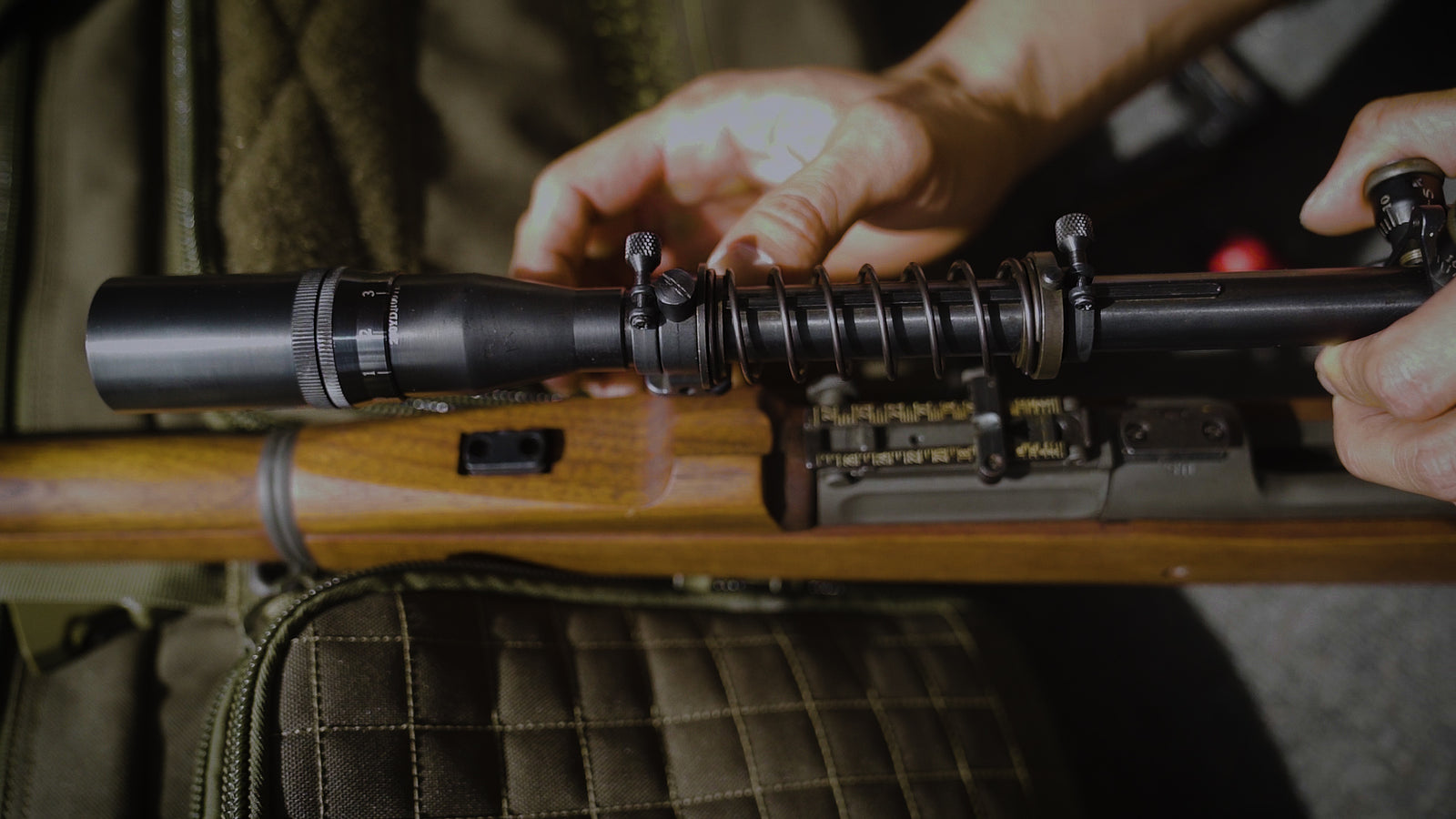This photograph captures a detailed close-up of a rifle being outfitted with a black scope. The left end of the scope, which is larger in diameter, is prominent, while the scope itself tapers off to the right. Encircling the midpoint of the scope is a silver spring, flanked by small screw-like projections for tension adjustment. The photograph prominently features a person's hands—his left hand is positioned at the right edge of the image, with his thumb resting over a component on the scope and his fingers cradling the cylinder underneath. His right hand, partially visible at the top right corner, helps steady the scope, with his thumb and fingers gripping it near the top.

The rifle itself exhibits a wooden body, with a light brown chamber area and some silver components, including what appears to be a bullet loading area. The wooden base of the rifle spans from the left center of the image towards the right, interspersed with gray mechanical parts on the right side. Below the rifle rests a greenish-gray backpack, identifiable by its zipper and sewn square pattern. In the background, the top left corner of the image shows out-of-focus green and gray material extending off the photo, adding context to the setting.